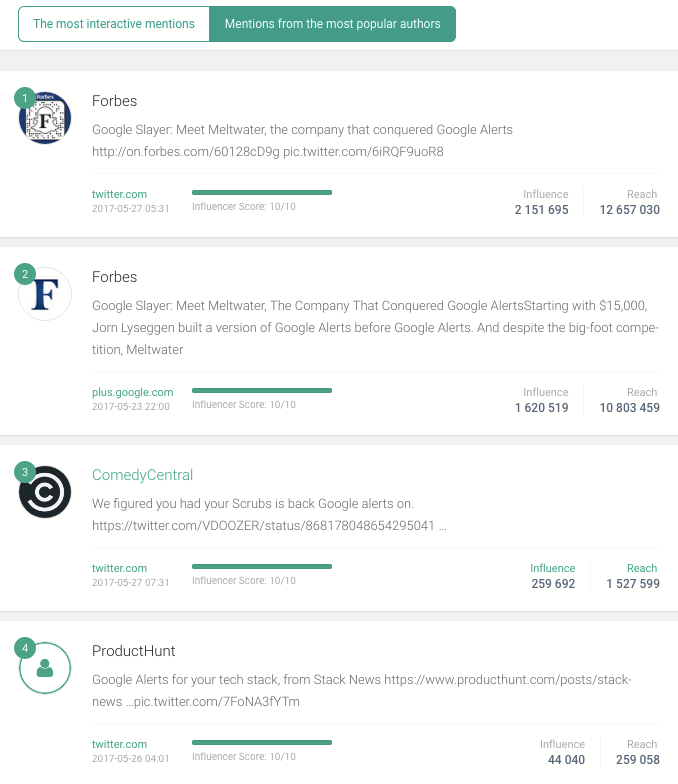The image, set against a white background, showcases a web page divided into several distinctive sections. In the upper left corner, a white box contains green text reading "The Most Interactive Mentions." This box is connected to another green box with white text labeled "Mentions from the Most Popular Authors."

Below these headers, the content begins with the first box featuring an excerpt from Forbes titled "Google Slayer: Meet Meltwater, the Company That Conquered Google Alerts," accompanied by a URL: http://on.forbes.com. Following this, the text references Twitter with the date "2017 527, 531" and mentions an "Influencer Score: 10 out of 10," along with another metric "Influence: 2 151 695."

Directly under this, the second box continues with another Forbes excerpt: "Google Slayer: Meet Meltwater, the Company That Conquered Google Alerts Starting with $15,000. Jorn Lissagen built a version of Google Alerts before Google Alerts, and despite the Bigfoot competition, Meltwater." Below this text, the Influencer Score reappears, noting "10 out of 10."

Each box and piece of text is neatly organized, providing a visual hierarchy that helps in digesting the information clearly.